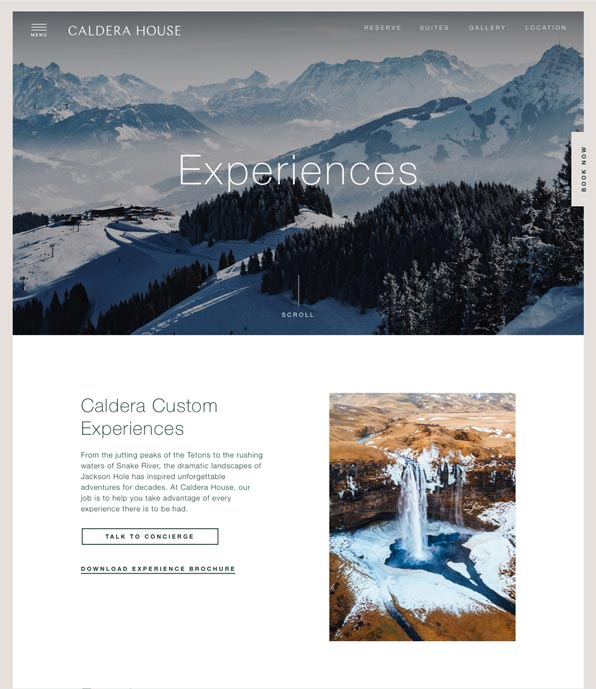The image displays the top section of a travel website for "Caldera House," featuring breath-taking views of a mountainous region. Prominently placed in the top left corner, the site's name "Caldera House" is accompanied by a three-bar menu icon, likely providing navigation to sections such as "Reserve," "Suitor," "Gallery," "Location," and "Caldera Custom Experiences." The words "Experiences" are emblazoned across the image, highlighting the adventure-focused aspect of the site.

In the upper half of the frame, towering mountains and lush greenery set a captivating backdrop, evoking a sense of exploration and natural beauty. Just below it, the website displays a text paragraph, possibly giving more details about the experiences offered. A secondary image of a majestic waterfall also suggests that the site is designed to inspire travel and discovery.

The lower half of the display features a clean, white background which contrasts crisply with the vibrant nature scene above. At the bottom, an image carousel indicator comprises five dots, implying the presence of multiple images that users can scroll through to get a fuller sense of the offerings. This carousel enhances the user experience by showcasing various scenic highlights Caldera House has to offer.